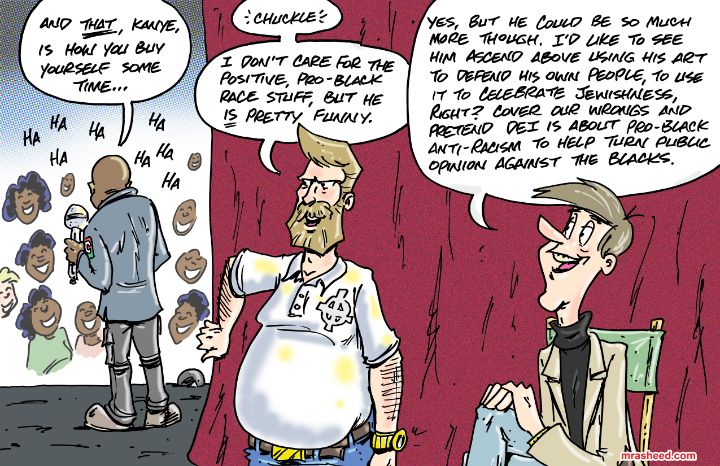The image is a hand-drawn comic strip split into two panels. On the left, an African-American comedian is seen on stage with his back to the viewer, addressing an audience. His speech bubble reads, "And that, Kanye, is how you buy yourself some time." The audience is depicted laughing at his joke. To the right, behind the curtain, there are two Caucasian men engaged in a conversation about the comedian. The man in the center, wearing a white shirt with a cross and circle symbol, has yellow stains on it and a watch on his arm. His speech bubble says, "Chuckle. I don't care for the positive pro-black race stuff, but he is pretty funny." The man to the far right, who is sitting in a director's chair and wearing a black turtleneck under a tan blazer, replies, "Yes, but he could be so much more though. I'd like to see him ascend above using his art to defend his own people, to use it to celebrate Jewishness, right? Cover our wrongs and pretend this is about pro-black anti-racism to help turn public opinion against the blacks." The curtain between them is red, adding a sharp contrast to the scene, and the comic is annotated with "marsheed.com."